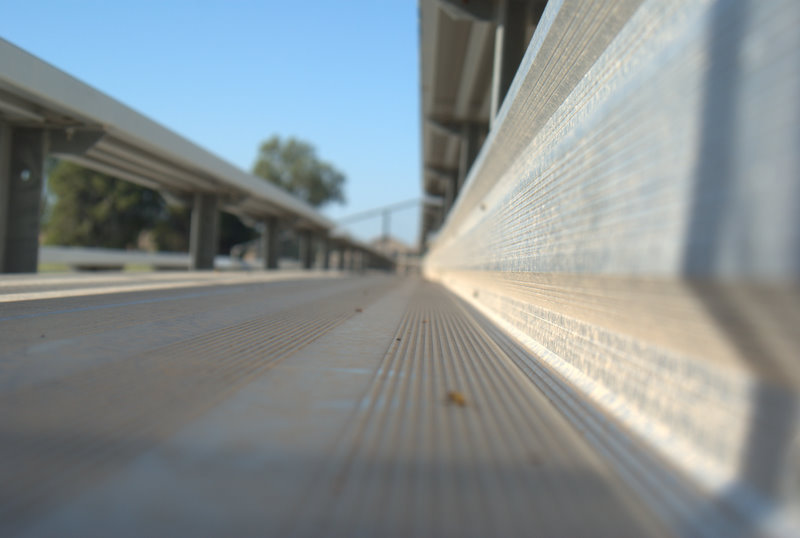In this image, the camera is positioned flat against one of the steps of outdoor bleachers, capturing a unique and surreal perspective. The bleachers are composed of long, slightly dirty, metallic boards supported by poles, typical of an athletic field or school stadium. The primary objects, including the bench extending directly through the center of the image, draw the viewer's eye along the length of the bleacher steps, which recede into the background from the top right to the bottom left. The blurred background reveals a backdrop of trees with green leaves and possibly another set of bleachers or a bridge in the distance. The sky is a clear light blue, and the sunlight casts long shadows, suggesting it's late in the evening. The colors predominantly observed are light blue, green, gray, dark gray, brown, and white, with no text visible. The setting is clearly outdoors, capturing a moment of stillness in what appears to be a well-worn but tranquil venue.